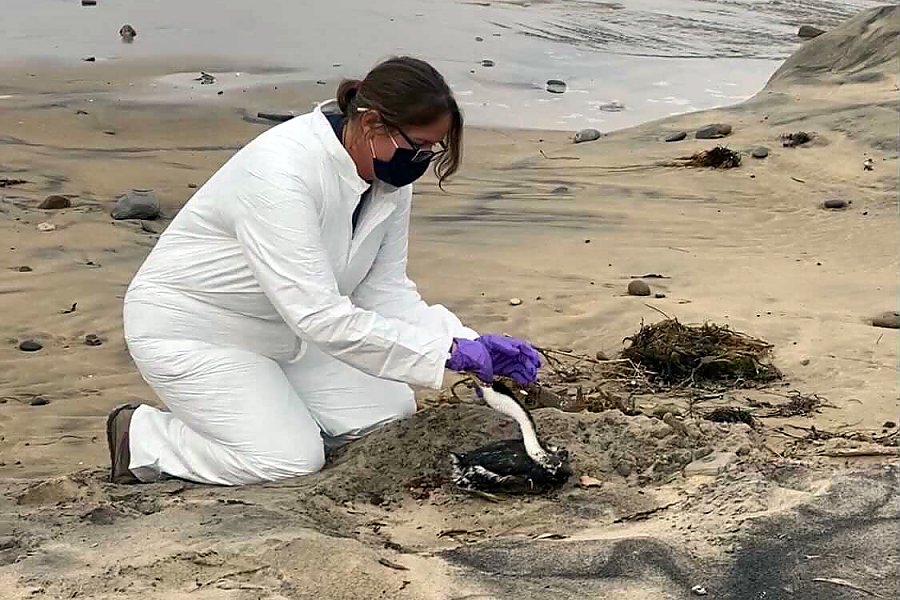In this striking beach scene, a woman dressed in a full white protective oversuit, resembling either a crime scene analyst or a scientist, is intently focused on an injured black and white bird. The woman, who has her black hair neatly pulled back into a bun, is equipped with purple nylon gloves, black glasses, and a black face mask covering her nose and mouth. She kneels on the wet, tan sand, which is littered with seaweed, rocks, and other debris scattered about. The waters, tinted brown and advancing onto the beach, add to the disarray of the scene. The injured bird, possibly a seagull or duck, appears dirty and distressed, as if it has been contaminated by oil. The woman is carefully examining and perhaps attempting to free the bird from entanglement, showcasing a tender moment of rescue amidst the chaos of a polluted shoreline.